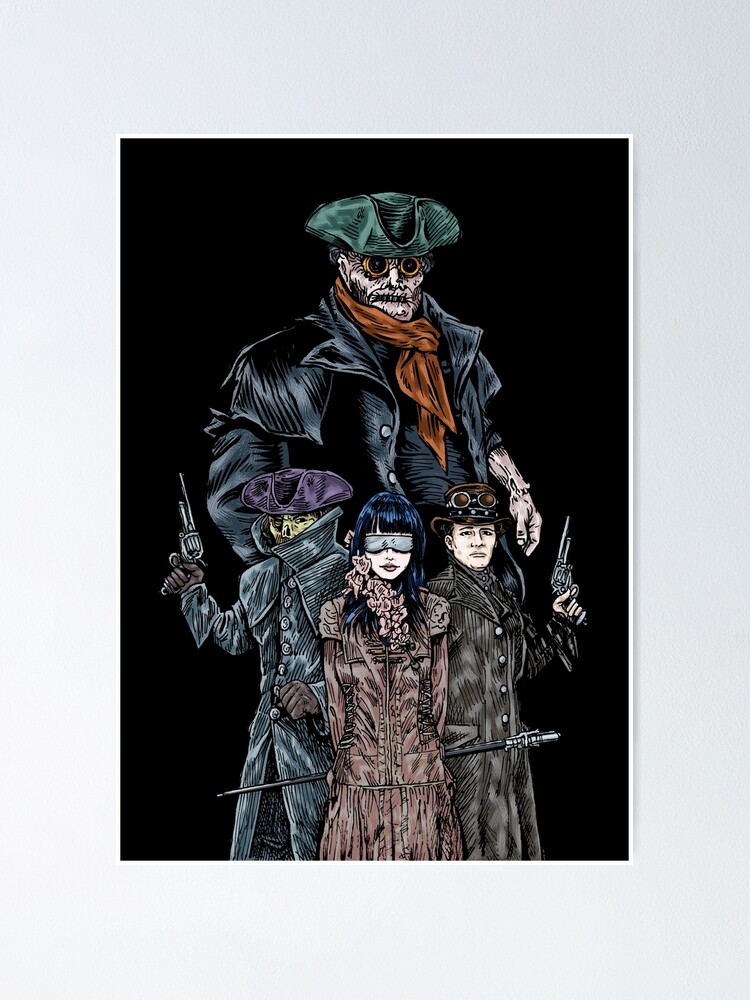In this visually striking painting framed by a pure white border, the centerpiece is a large, foreboding figure with an ancient, wrinkled face and piercing orange eyes. He is dressed in a dark-colored jacket and shirt, complemented by an armored scarf around his neck and a green tri-corner hat perched atop his head. This imposing character, reminiscent of an eerie pirate or ghostly figure, dominates the mostly black background of the painting.

Beneath this central figure are three smaller characters, each distinct in their appearance and attire. At the center stands a woman with strikingly blue-black hair, styled to look almost like a midnight hue, wearing glasses and a brownish jacket. Behind her back, she wields a sword. To her left, a figure clad in a light gray jacket and purple hat holds a gun, his face an unusual green hue, accentuated by gloves on his hands. To her right is another man, dressed in a different shade of brown jacket, also holding a gun. This man sports a top hat and glasses perched on top of it. The trio contrasts sharply against the dark figure looming above them, adding depth and storytelling to the artwork, which is set against a white-framed border, enhancing the ominous yet intriguing scene.